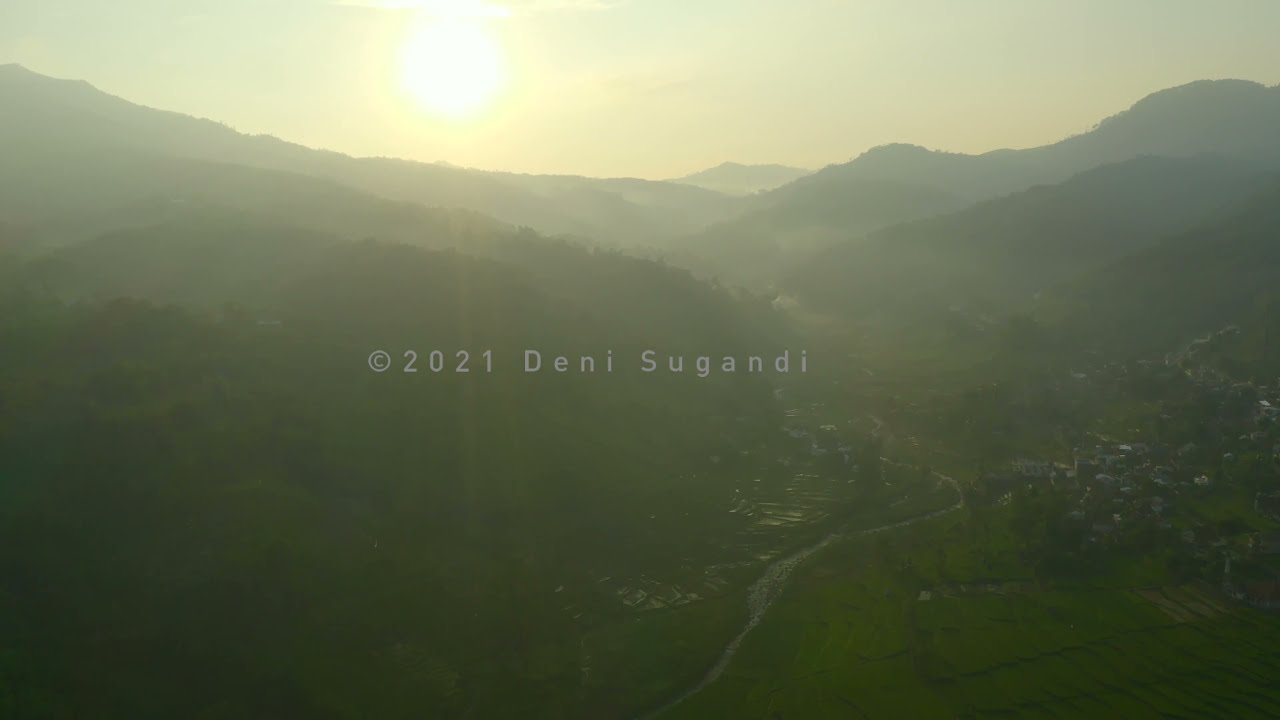This photograph captures an expansive aerial view of rolling, green mountains and lush hills filled with vibrant vegetation, including trees, grass, and bushes. In the bottom right corner, a small, hazy village or town is visible, with dark-colored (likely black or gray) buildings clustered along the banks of a creek. The landscape features a long road that meanders through the greenery. The bright, radiant sun, possibly hinting at dawn with its intense white center transitioning to a soft yellow, dominates the upper right portion of the sky, casting a golden hue over the scene and some hilltops. The varying heights of the mountains give the image a sense of depth and scale. Despite the brightness of the sun, the photo appears somewhat hazy, lending a shadowy yellow tint throughout. Additionally, there's a copyright symbol and gray text in the center of the image, reading "© 2021 Denny Sugandhi."